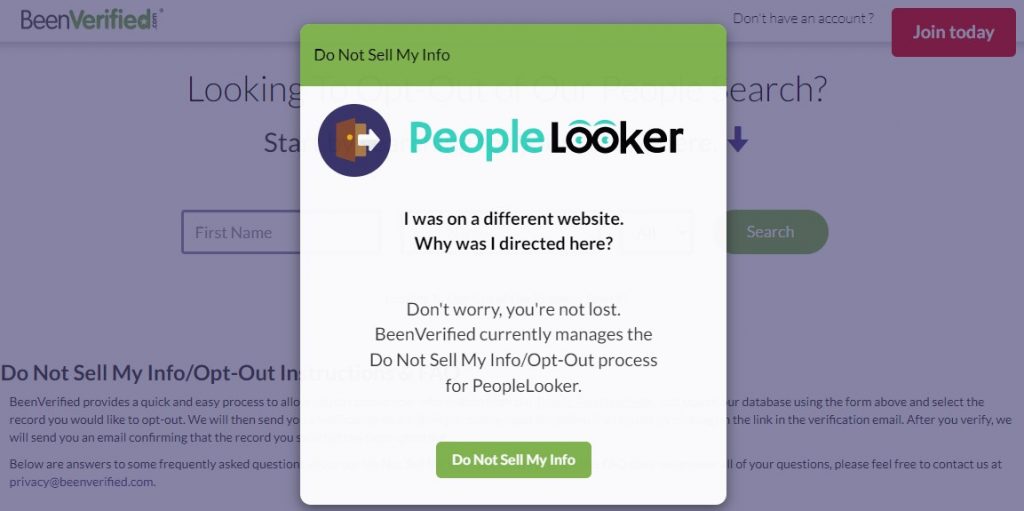Screenshot of a web page featuring a white and green pop-up window superimposed on a muted gray-toned background. The background window displays partially visible information. In the top left corner of the background, the header reads "Been Verified" in green text. The upper right corner features a prominent red rectangular button labeled "Join Today." To the left of the pop-up, there is a visible portion of a text box with the placeholder "First Name," alongside a green oval button labeled "Search" in white text.

At the bottom left of the background, bolded black text reads "Do Not Sell My Info / Opt Out," accompanied by a paragraph of detailed information.

The main pop-up window has a green bar across the top with "Do Not Sell My Info" written in black on the left side. The pop-up's main section has a white background. A large icon on the left side depicts a dark circle with a brown open door and a white arrow pointing at the green word "People." Next to it is the word "Looker" in black, with the letters 'o' styled as blue dot eyes and green arches above them resembling eyebrows.

Centrally positioned black text on the pop-up reads, "I was on a different website. Why was I directed here?" followed by reassuring text: "Don't worry. You're not lost. Been Verified currently manages the Do Not Sell My Info / Opt Out process for PeopleLooker."

The pop-up concludes with a horizontal green bar at the bottom, displaying "Do Not Sell My Info" in white text.